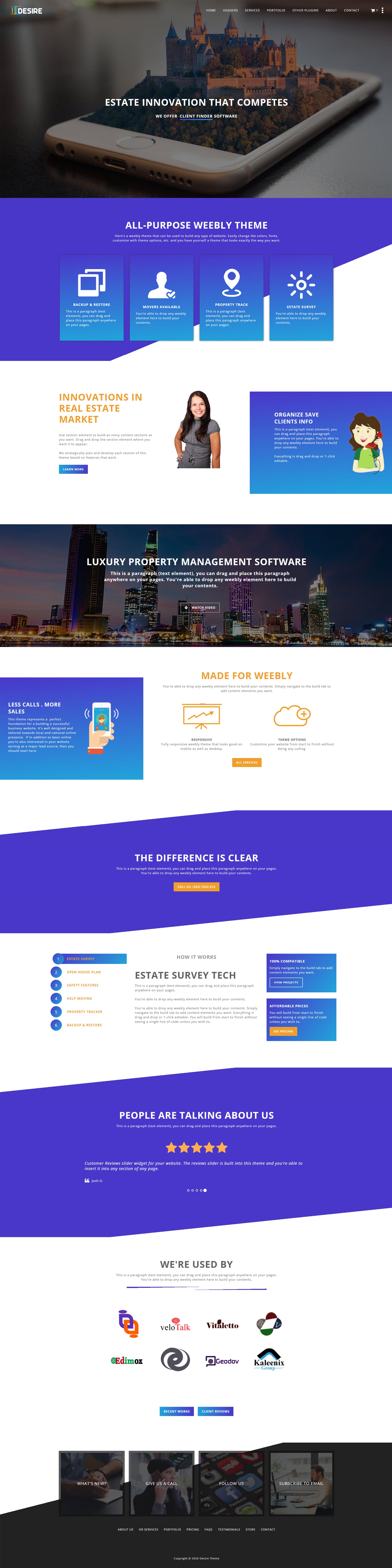This image is a detailed screenshot of a webpage, displayed on a larger background to facilitate scrolling. 

At the very top, the screenshot captures standard cell phone icons including signal bars and battery percentage indicators at the upper left and right corners respectively. These elements are notably tiny, hinting that the original screenshot has been scaled down to fit into a specific banner size.

Dominating the top section of the webpage, there is a captivating background image featuring an iPad placed on a table. Emerging from the top of the iPad in a 3D effect is a city skyline. Overlaid on this image is a title in bold text that reads "Estate Innovation That Competes," followed by a line of smaller text underneath.

Directly below this image, there is a prominent blue banner with very small white text, though the exact message is not discernible. Below this banner, four icons are displayed sequentially: a pair of photos, a stick figure, a location pin, and a lightbulb.

Continuing down the page, there is a smaller white banner featuring the image of a woman on the right. This banner is headed by a title in red letters, accompanied by smaller blue text underneath. Adjacent to this, on the right side, is a blue box containing a clipart image of a woman along with small white text.

The central portion of the webpage showcases a visually striking banner with a city skyline in the background. Overlaid on this image, in small white letters, is the phrase "Luxury Property Management Software," followed by descriptive text.

On the bottom left side, a small blue banner features a clipart icon of a cell phone, with descriptive text positioned to the left of the icon. Finally, at the very bottom of the webpage, there is a box filled with various logos, indicating affiliated brands or partners.